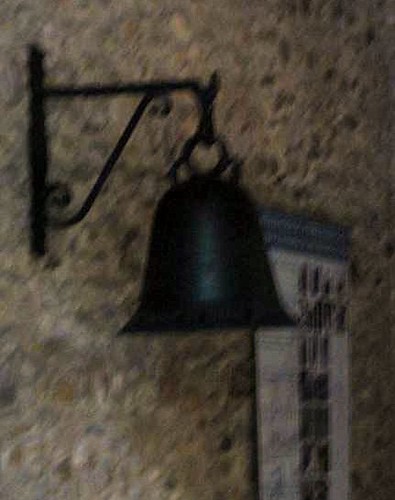The image depicts a black bell mounted to a granite, brownish multi-colored wall, connected by a metal bracket with a line structure featuring two squiggly supports. The focal point of the picture is the bell, which is situated centrally with a small circular piece at its top attaching it to the bracket. In the background, towards the bottom right, there is a sign or calendar that is predominantly white with blue at the top, but the entire image is highly out of focus, rendering the text and finer details indistinct.